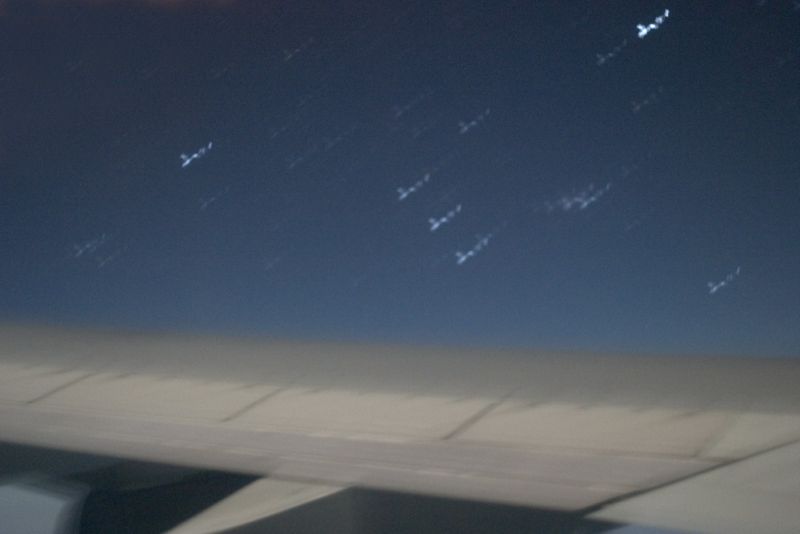The image is a blurry and abstract close-up view of an airplane wing against a dark blue sky. The sky gradually fades into a slightly lighter blue toward the horizon, occupying about two-thirds of the upper part of the image. Strewn across this part of the sky are numerous white streaks that give an impression of motion, some diagonal in orientation, pointing towards the lower left-hand corner. The bottom third of the image features a flat, metal-lined object in shades of gray and beige, resembling the aircraft wing that stretches from left to right across the frame. The wing includes a triangular point that extends forward into the image, and the section nearest to the viewer has a darker gray tone transitioning to lighter hues. Overall, the entire photograph appears to be taken in landscape format and is notably low in detail due to its blurry focus.